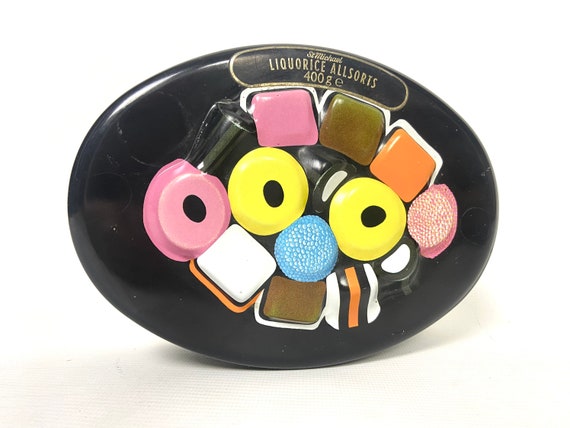The image showcases a small, antique, black, oval-shaped container, likely made of plastic, designed to hold licorice candies. The container is labeled "St. Mikan Licorice Allsorts" in gold lettering, with a weight indication of 400 grams, denoted as '400G E'. The top of the container features a prominent oval label with ornate lettering curved around it. The front of the container is adorned with a colorful, intricate depiction of various licorice candies, arranged in a somewhat layered manner. The depicted assortment includes square licorice pieces in pink, brown, and orange, as well as round ones featuring black centers in yellow and pink hues. Notably, there's a distinctive striped licorice in white, black, and orange, a blue round licorice with dotted white candies, alongside other pieces in shades of black, yellow, and brown. The overall background of the image is completely white, making the details on the container stand out vividly.